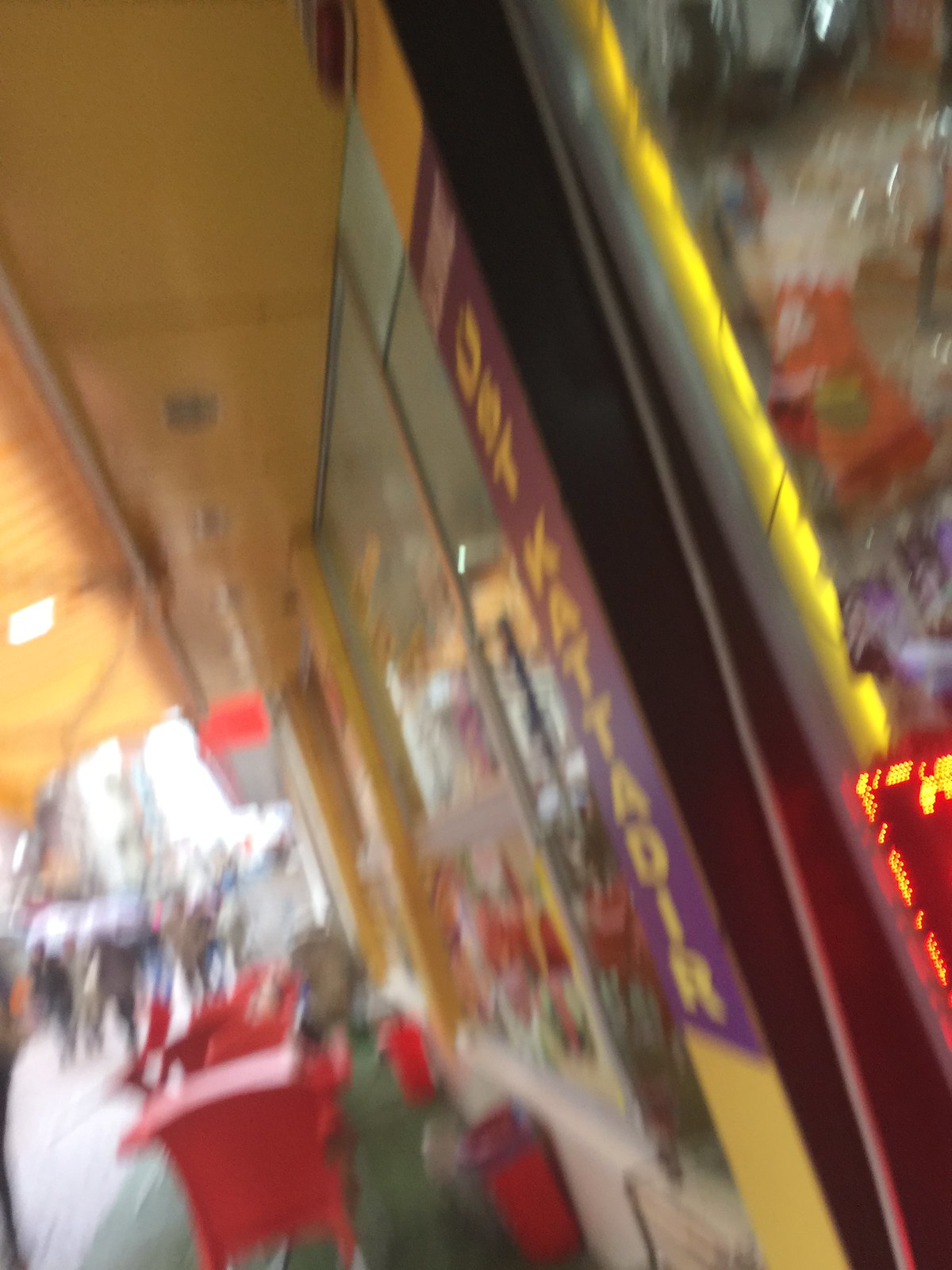The image captures a lively storefront scene from the sidewalk, dominated by a blurred ambiance as if snapped hurriedly while walking past. The storefront is painted yellow, complemented by a purple, likely foreign, sign that reads "USTKATTADIR," positioned between windows and the doorway. The angle of the photograph is slightly tilted to the left by around 20 to 30 degrees, adding to the disorienting effect of the blur. Under a yellow awning, the scene is dimly lit, contributing to a desaturated and overcast mood. Display windows are adorned with various decorations, including hints of red and green, typical of festive decor such as a red Christmas stocking. Below the awning, a red chair or possibly a wagon is faintly visible. Silhouettes of people, approximately 20, are discernible in the distance, walking along the street, adding to the bustling street atmosphere. The combination of these vibrant elements produces a chaotic yet vibrant snapshot of a bustling shopping area.